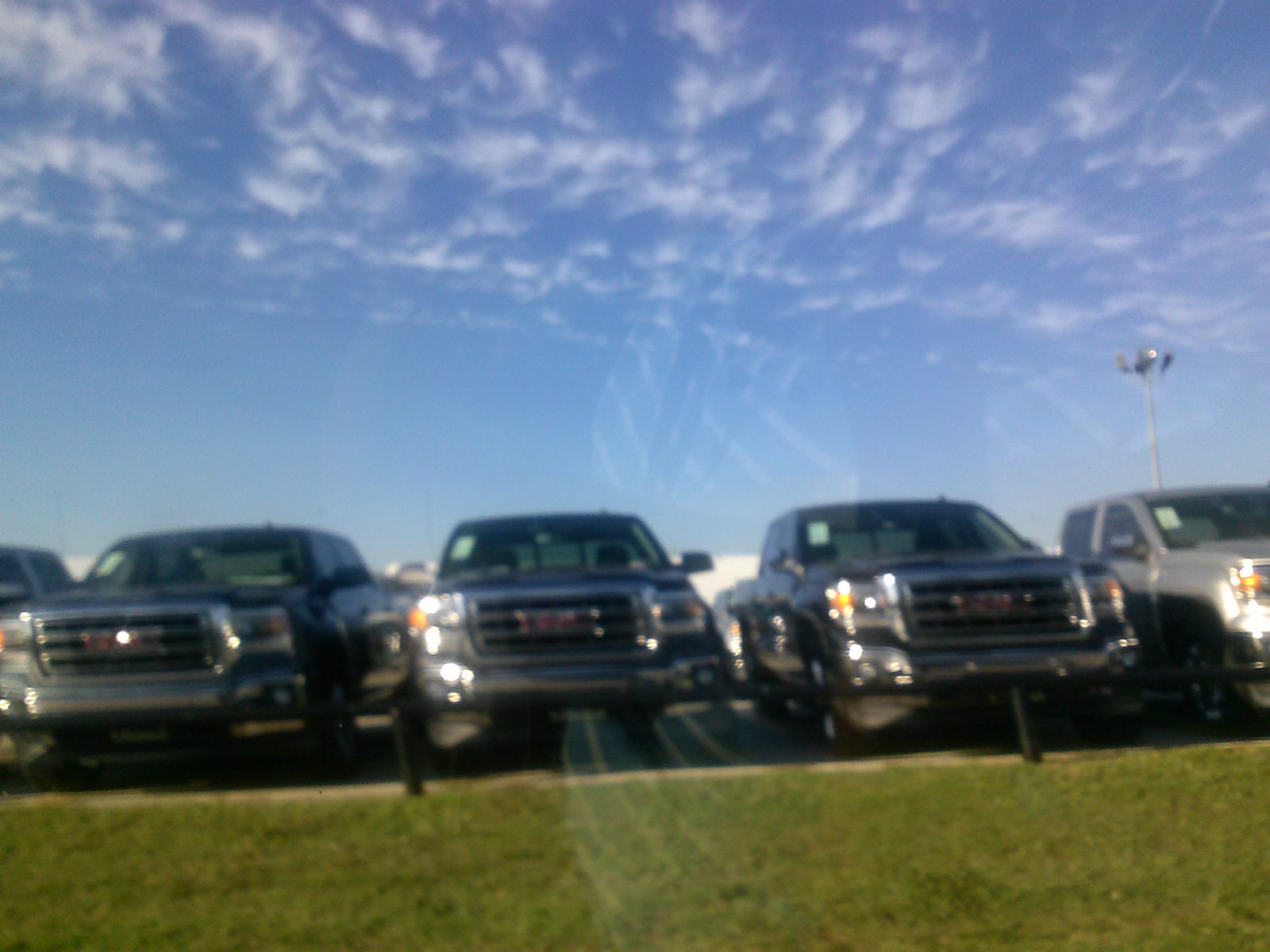The photograph depicts a slightly blurry scene of four trucks parked in a line, facing the camera. In the foreground, there’s a patch of green grass followed by a short black guardrail separating the grassy area from the parking lot where the trucks are situated. The trucks, which seem to be part of a dealership, feature silver grilles all adorned with the letters GMC in red. Starting from the left, the first truck is black with a wide grille. The second and third trucks are both blue, with the third one being almost identical to the second. Partially off-camera to the right is a silver truck, distinguishable by its two side windows and windshield. A piece of paper, likely indicating the price, is visible on the upper left-hand side of the windshields of each truck. Behind the trucks, the sky is brilliantly blue, dotted with fluffy white clouds, and a tall, seemingly lit street light stands in the background.